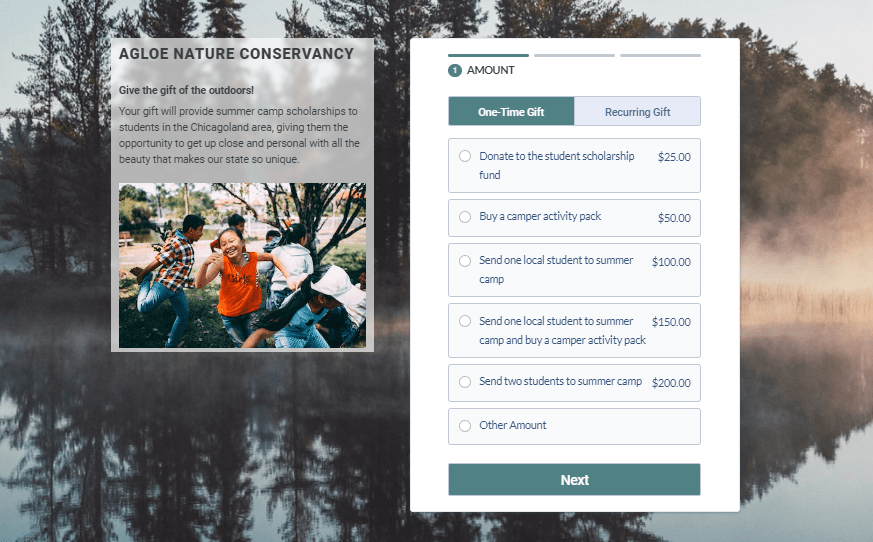A serene photograph depicts a tranquil scene of lush green trees mirrored in the calm, glassy surface of a lake. On the right side of the image, a gentle haze or smoke rises from the water, adding a mysterious and ethereal quality to the landscape. 

Superimposed on the image is a semi-transparent vertical rectangle, allowing a glimpse of the picturesque scenery behind it. The text within this rectangle reads: "AGLOE Nature Conservancy. Give the gift of the outdoors. Your gift will provide summer camp scholarships to students in the Chicagoland area, giving them the opportunity to get up close and personal with all the beauty that makes our state so unique." 

Accompanying this message is a photograph of children joyfully playing, encapsulating the essence of the camp experience. Below the text, donation options are presented with corresponding amounts and descriptions: 
- Donate to the student scholarship fund, $25.
- Buy a camper activity pack, $50.
- Send one local student to summer camp, $100.
- Send one local student to summer camp and buy a camper activity pack, $150.
- Send two students to summer camp, $200.
- Other amount.

Donors can choose between a one-time gift or a recurring contribution using the provided toggles. A progress bar indicates the current donation amount, encouraging further contributions.